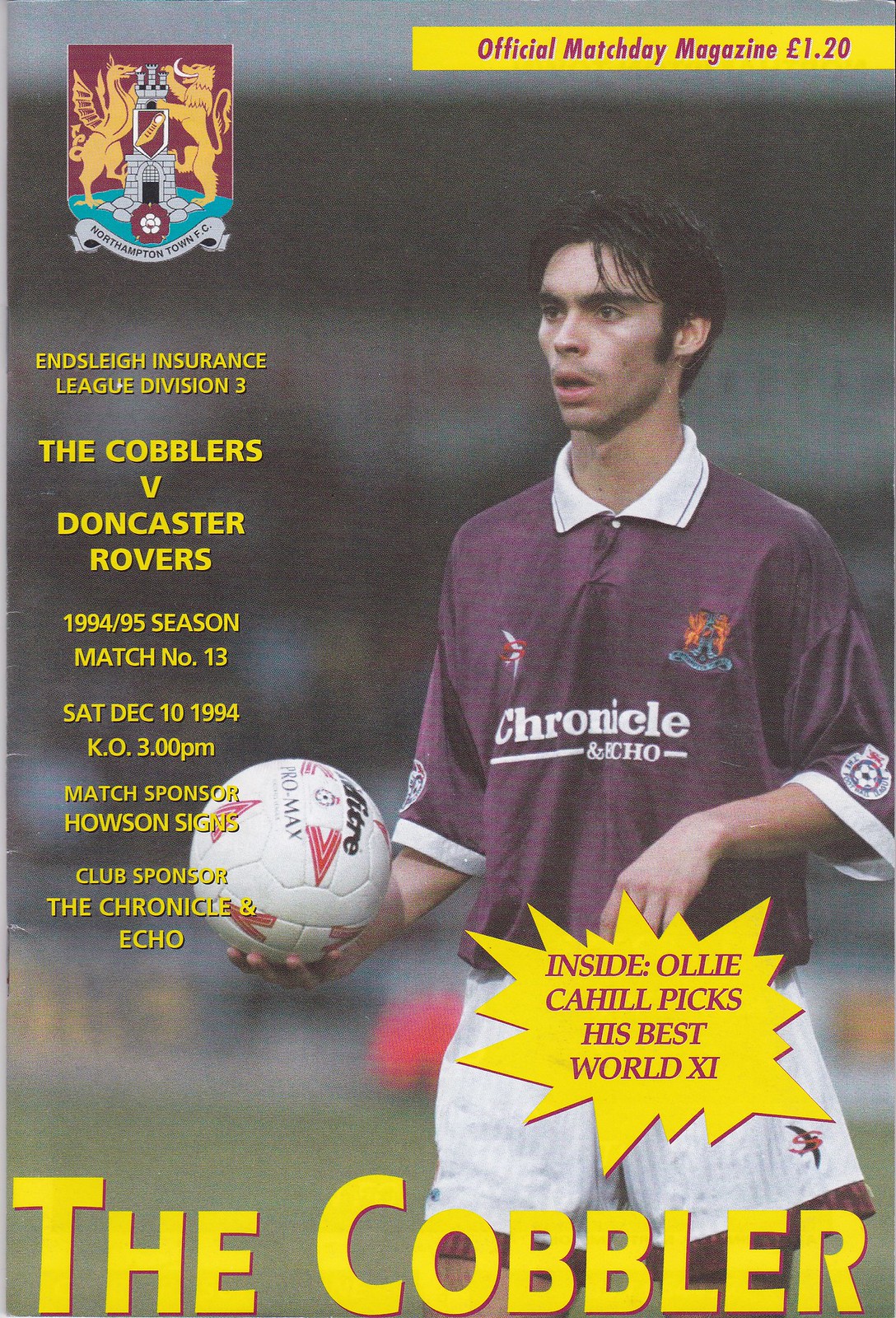The image is a detailed cover of an official match day magazine priced at £1.20. Dominating the center is a young man wearing a dark purple soccer jersey with "Chronicle" emblazoned across the chest, holding a soccer ball. Below him, a large yellow burst highlights an inside feature titled "Ali Cahill Picks His Best World XI." On the left side of the cover, text in yellow declares "Endless Insurance League Division 3: The Cobblers vs. Doncaster Rovers, 1994-95 Season, Match No. 13, Saturday, December 10th, 1994, K.O. 3 p.m., Match Sponsor: House and Signs, Club Sponsor: The Chronicle & Echo." Prominently at the bottom, in bold white letters, it states "The Cobbler."